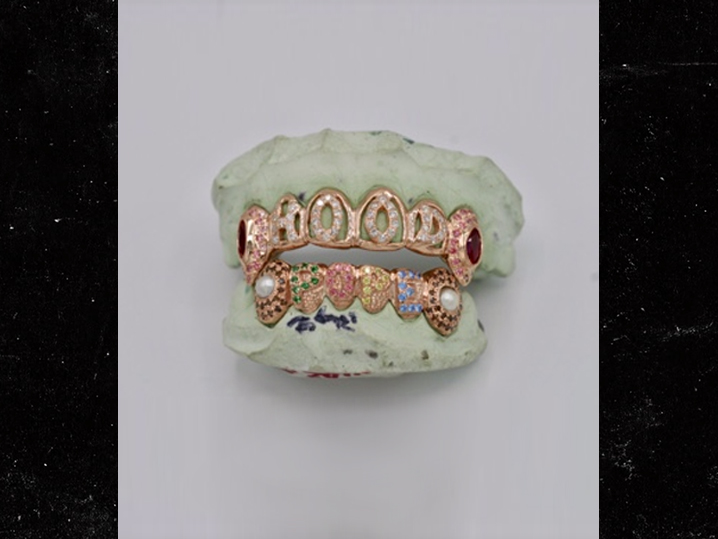This image features a striking piece of artwork displayed against a subtle gray background. It depicts a set of dentures crafted from what seems to be green plaster that mimics the appearance of gums. The "teeth" are fashioned from a coppery, shiny metal and are intricately outlined, enhancing their standout appearance. Adorning these metal teeth are an array of sparkling gems and pearls. In particular, the top section showcases white or clear diamonds, while the bottom section reveals colorful gems—specifically, a pattern of a yellow 'P', red 'O', green 'P', yellow 'O', red 'O', yellow 'P', and blue 'E' spelling out "P-O-P-E." Below these letters, a signature-like black marking can be observed. The overall effect is reminiscent of an elaborate rapper's grill, combining elements of luxury and modern artistry.